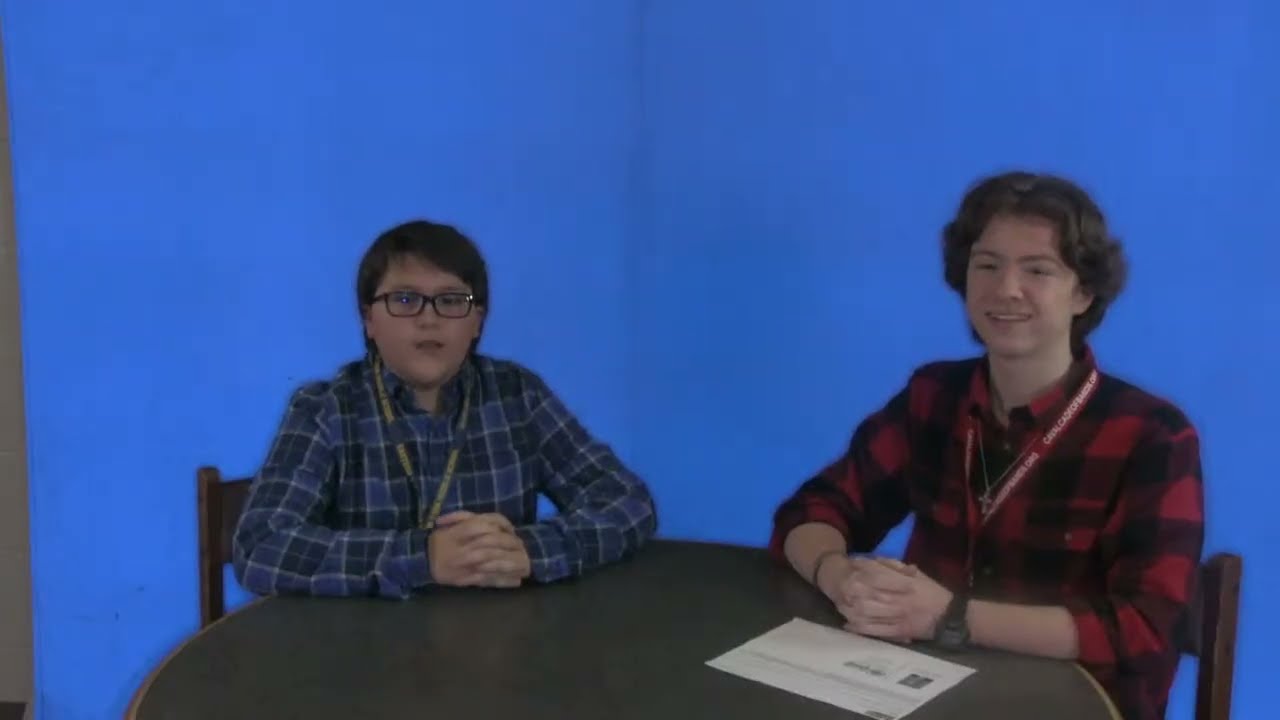In this image, we see two men seated at a round, dark gray table, which is centered at the bottom of the photograph. Each man is positioned slightly towards the sides; one to the left and one to the right of the image. The backdrop is a solid, bright blue that appears to be either a wall or a curtain, suggesting an indoor setting, possibly a personal or informal space such as a kitchen.

The man on the left is wearing a blue and dark blue plaid flannel shirt. He has dark hair parted to the right, wears dark glasses with black frames, and is slightly chubbier in build. A blue lanyard with yellow text hangs around his neck. His hands are folded on the table before him.

The man on the right sports a red and black plaid flannel shirt with a red lanyard around his neck and a silver chain with a cross. He has brown hair that curls slightly at the ends, and he too has his hands interlaced on the table. Both men sit in dark-colored chairs that appear to be wooden.

On the table, in front of the man on the left, lies a single sheet of white paper. The overall feel of the image suggests it is a personal photograph, potentially taken by a family member, capturing a moment between two individuals in a casual setting.